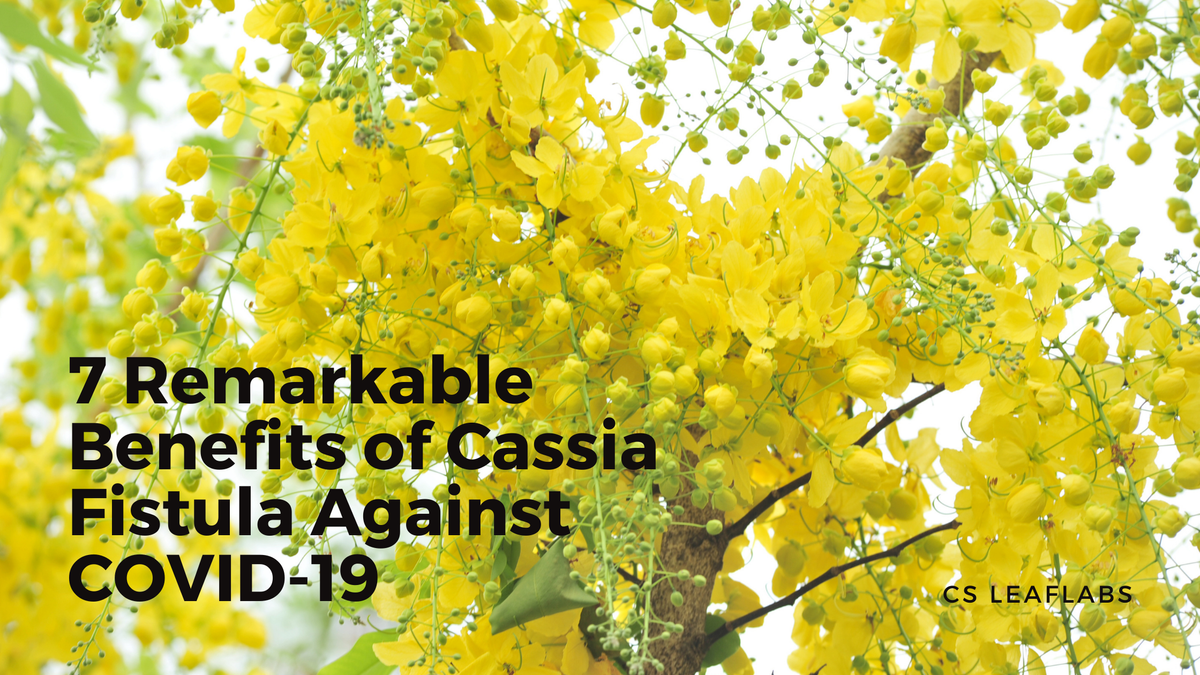The image captures a vibrant outdoor scene dominated by a Cassia fistula tree, whose branches are adorned with clusters of small yellow bell-shaped flowers and interspersed with green leaves. The bright, white, cloudy sky provides a striking backdrop to the tree’s verdant and floral display. A prominent branch extends from the bottom center of the image toward the upper right, laden with yellow flowers, some still in bud form while others are fully bloomed. Additionally, several thinner branches fan out, dotted with seeds and spiky green offshoots. Text in the lower corners of the image enhances its informative nature: in bold black font on the lower left, it reads "Seven Remarkable Benefits of Cassia Fistula Against COVID-19," and in smaller black print on the lower right, it says "CS Leaf Labs." The overall scene is one of natural beauty intertwined with educational messaging about the potential health benefits of this flowering tree.